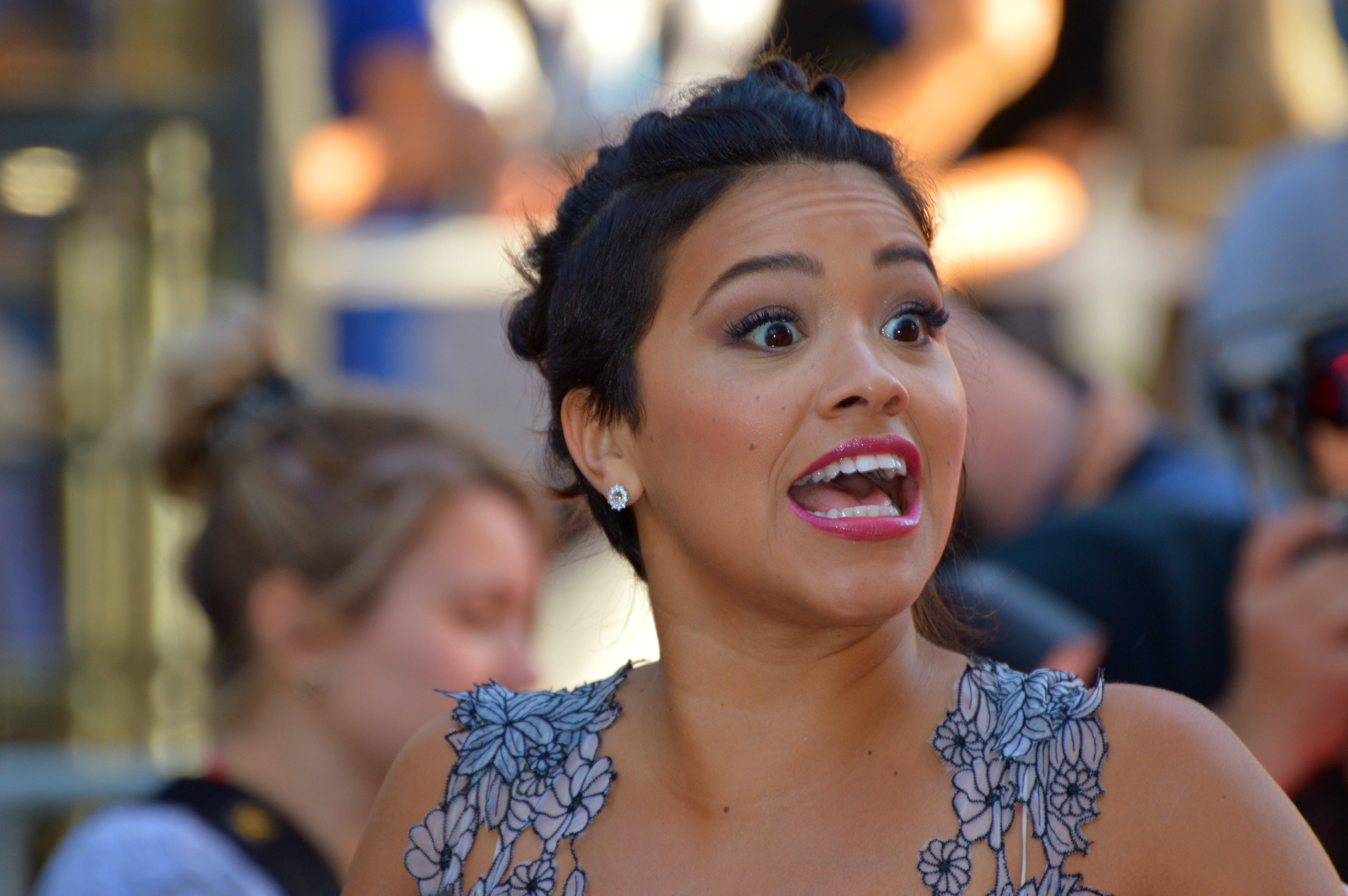The image captures a close-up of a fair-skinned woman with short, very dark hair, styled with the sides closely trimmed and the top pulled back into a braid. She is facing slightly to her left with her mouth open, which suggests she might be yelling, singing, or surprised. She has dark, well-defined eyebrows, thick dark lashes, and dark eyes. Her makeup is meticulously done, featuring bright red lipstick. She is adorned with a silver earring in the one visible ear. She wears a sleeveless top with floral-patterned straps in white and blue, visible above her bosom. The blurred background reveals a blonde woman with her hair in a bun and multiple other indistinct figures, including a man pointing what appears to be a camera. The setting is brightly lit, making all the details clear.